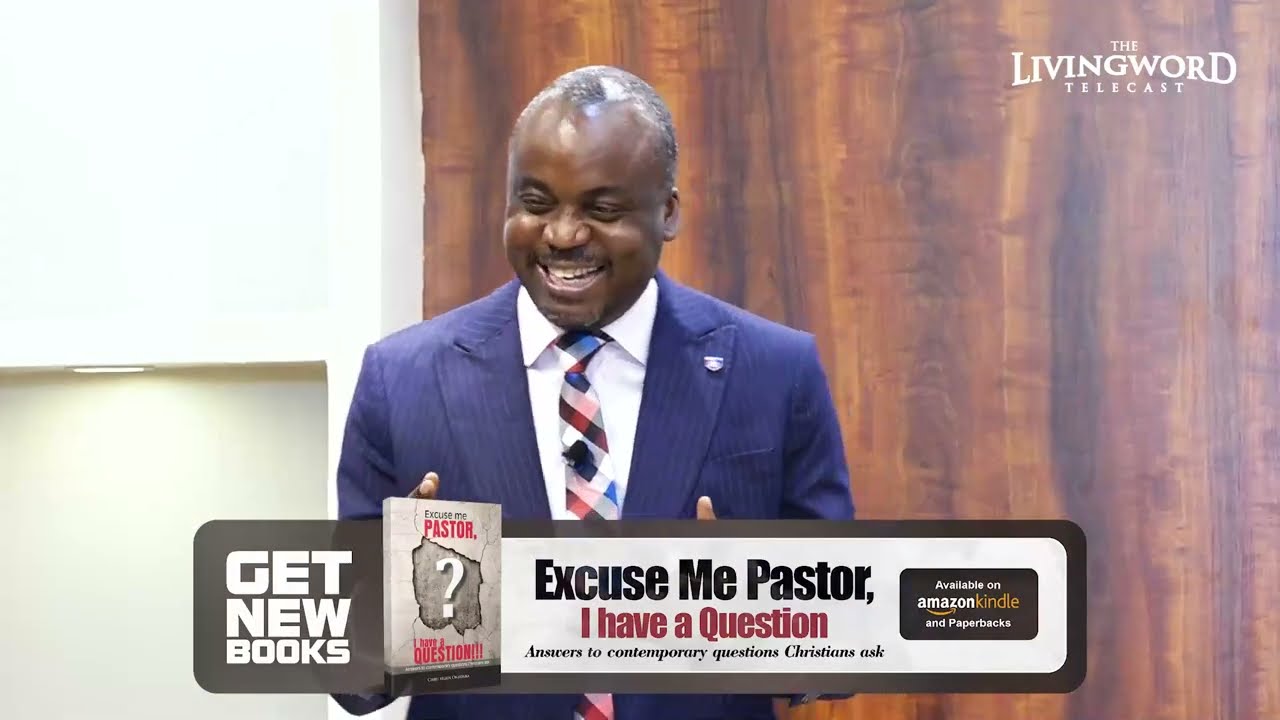The image is a landscape-oriented color photograph capturing an African-American man speaking against a wood-paneled backdrop. He is depicted wearing a navy pinstripe suit with a white dress shirt and a plaid red, blue, and white tie. His hair is a short, salt-and-pepper style with a receding hairline, and he has a small goatee complemented by a thin mustache. The man is smiling broadly, causing his eyes to squint, and he appears to be speaking in a joyous and animated manner.

Text on the upper right corner of the image reads "The Living Word Telecast" in all capital letters, indicating it is from a television broadcast. A banner runs across the bottom of the image promoting a book with the text "Get New Books" on the left side. Beside this text, there is an image of a book titled "Excuse Me, Pastor," followed by the subtitle "I Have a Question" in red text. Below this, in smaller black text, it states, "Answers to Contemporary Questions Christians Ask." To the right of the subtitle, the banner includes the Amazon Kindle logo, indicating the book's availability on Kindle and in paperback. The entire scene is set against a wood-paneled wall, emphasizing the formal and polished setting likely within a church or similar venue.